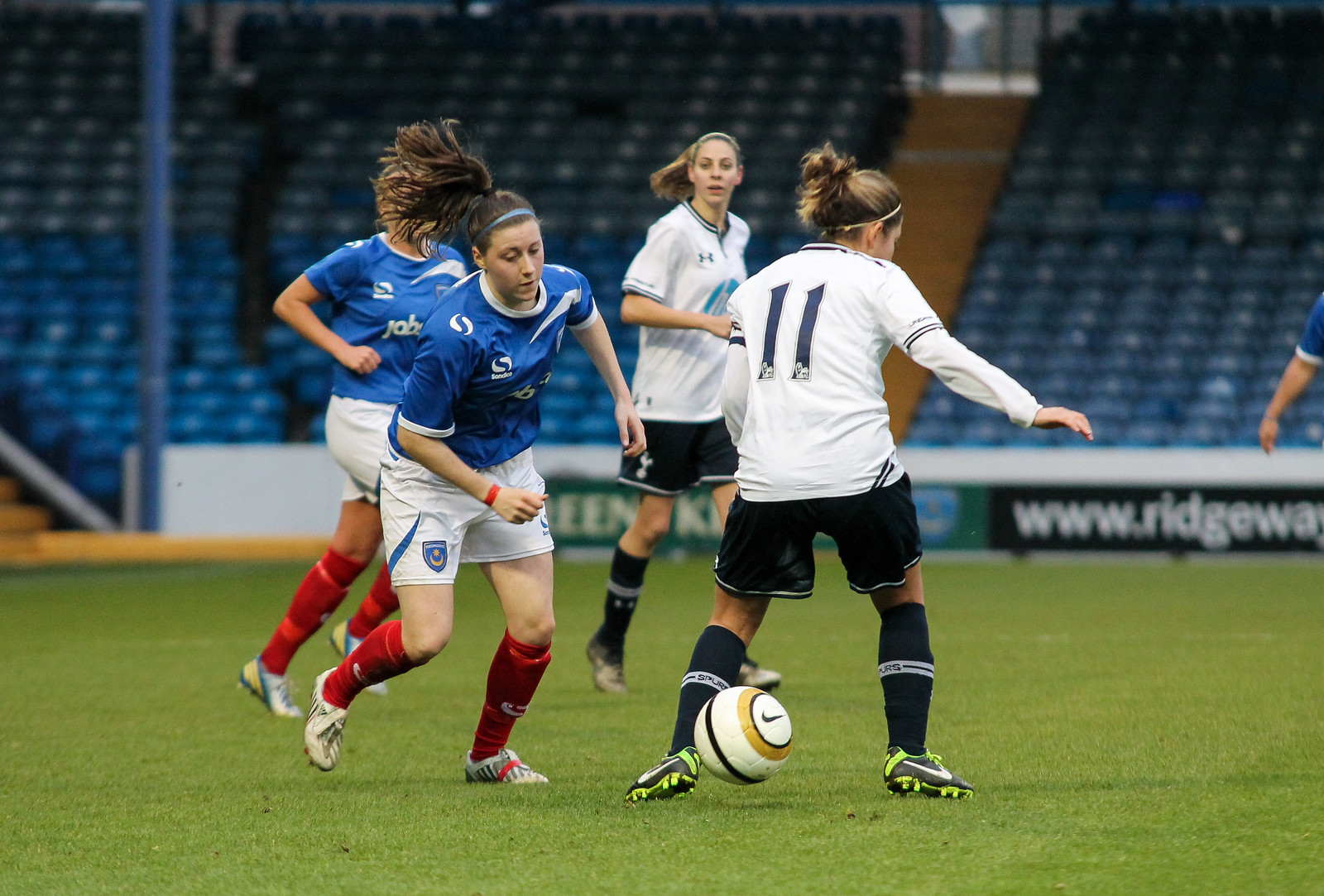In this dynamic photograph, four women are fiercely competing on a lush green field, intently focused on a white soccer ball at the center of their action. Two of the women are sporting white shirts paired with black shorts and long black socks, while the other two are clad in blue shirts, white shorts, and long red socks. The image captures the intensity as all four athletes go after the ball, embodying the spirit of the game. Surrounding the field are rows of blue seats in the stadium, sparsely occupied by spectators. The well-manicured grass suggests a professional playing environment. Though the exact weather conditions are unclear, it appears to be an outdoor event, with an ambiguous sky that could either indicate a sunny or overcast day. The scene exudes energy and competition, encapsulating a moment of high action in what could be a crucial play of the match.